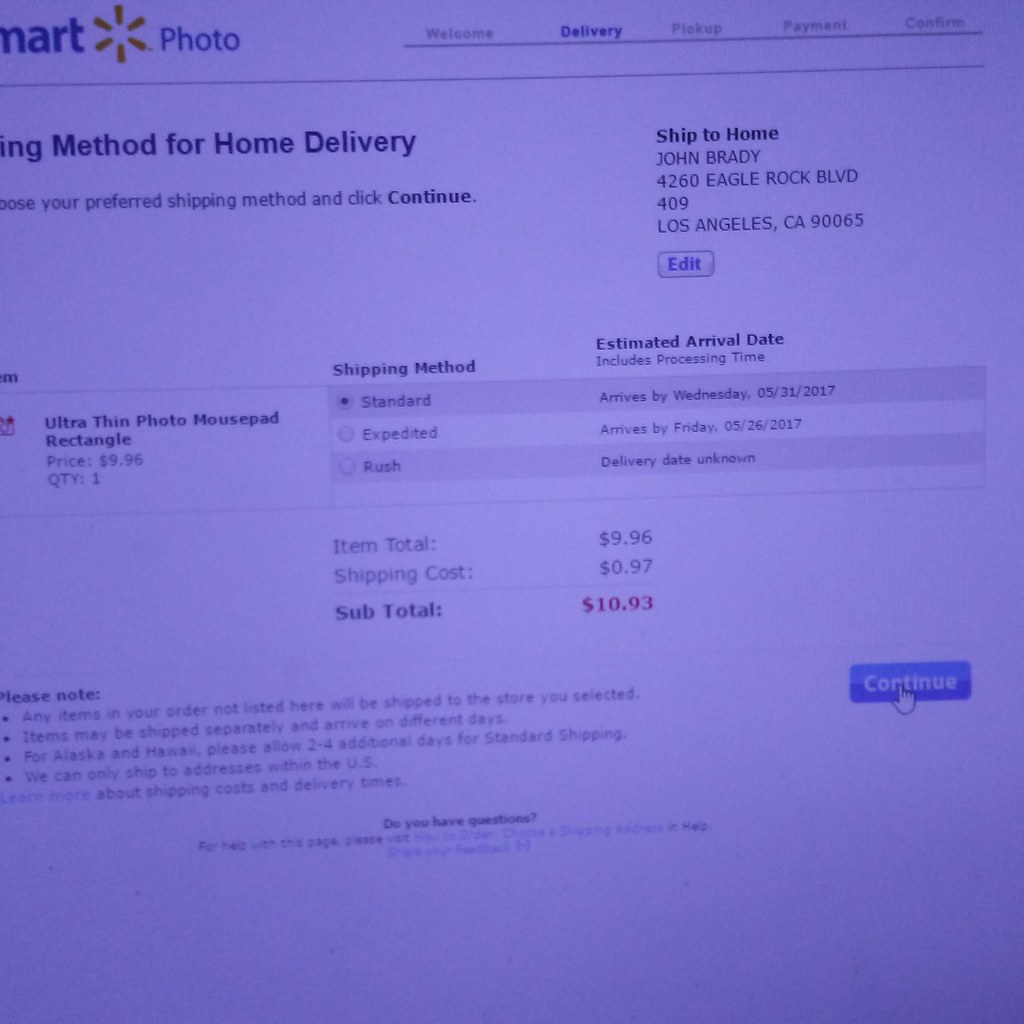A screenshot captures the checkout page from Walmart Photo. The screen displays a light purple tint despite being a white document, likely due to the computer monitor's settings. In the upper left corner of the image, parts of the Walmart logo are visible, with the blue "M" and "A-R-T" partially seen alongside the recognizable Walmart spark logo and the word "photo." The top right corner of the invoice shows that the order is set to be shipped to the client's home, identifying the shipping method as home delivery. Just below, the purchased item is detailed: an ultra-thin rectangular photo mouse pad. The standard shipping method is indicated, and the subtotal is listed as $10.93. In the lower right corner of the image, the "Continue" button is prominently displayed, with a white hand pointer icon hovering over it, ready to proceed with the purchase.